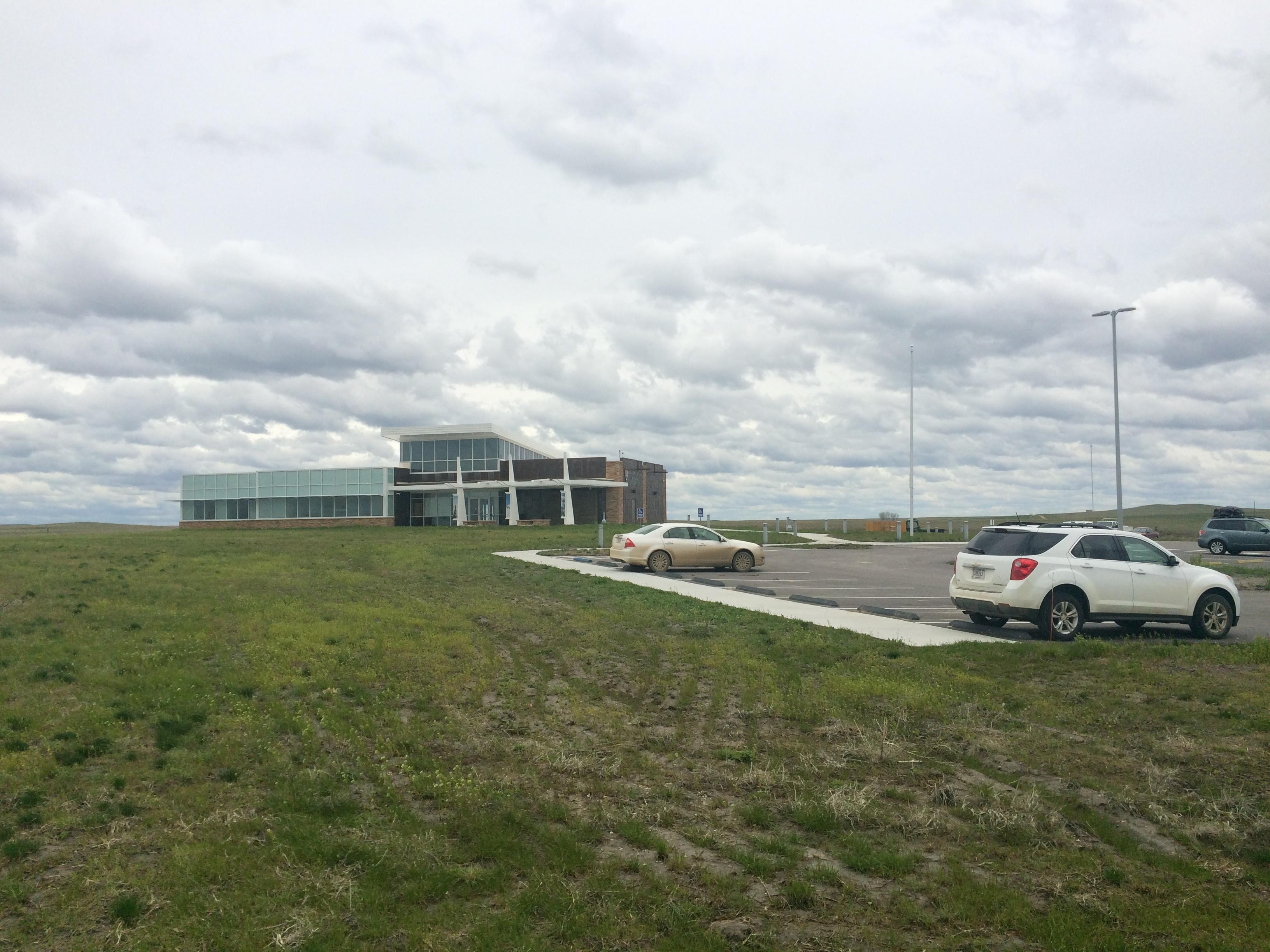The image depicts a modern, newly constructed glass and cement building with three prominent white pillars across the front, standing alone in an expansive, treeless landscape that resembles the Great Plains, possibly South Dakota. The sky occupies half of the photo, filled with gray, cumulus clouds that exhibit distinct shapes and forms. The building is set against a green field of grass, emphasizing its isolation. In the foreground, there is a small parking lot with about 20-30 spaces, featuring three visible cars: a white SUV in the foreground, a tan sedan, and another SUV parked farther away. Additionally, there are two electrical poles near the parking lot, adding to the stark and open atmosphere of the scene.